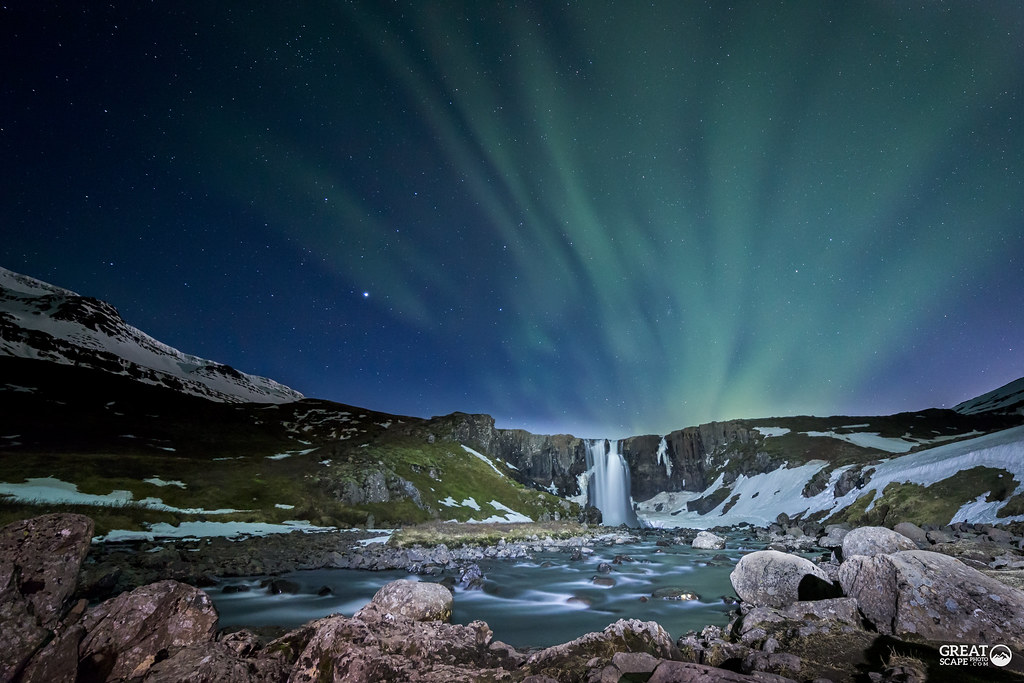The photograph depicts a breathtaking outdoor scene under a mesmerizing sky. The sky is awash with mid-green and turquoise lights that illuminate the landscape, contrasting beautifully with its indigo hue on the right and navy blue on the left. White speckles, representing stars, add a touch of celestial beauty. Below this radiant sky lies a rugged hilly area covered in green grass, with hints of rock and snow. Dominating the center is a majestic waterfall cascading down a cliff, feeding into a teal-colored body of water in the foreground. This pool is surrounded by numerous gray rocks, adding to the rugged charm of the scene. The rocky terrain stretches across the foreground, creating a natural frame for the water. To the right, a banner reads "greatscapephoto.com" in white text, accompanied by a circular logo featuring a white mountain.